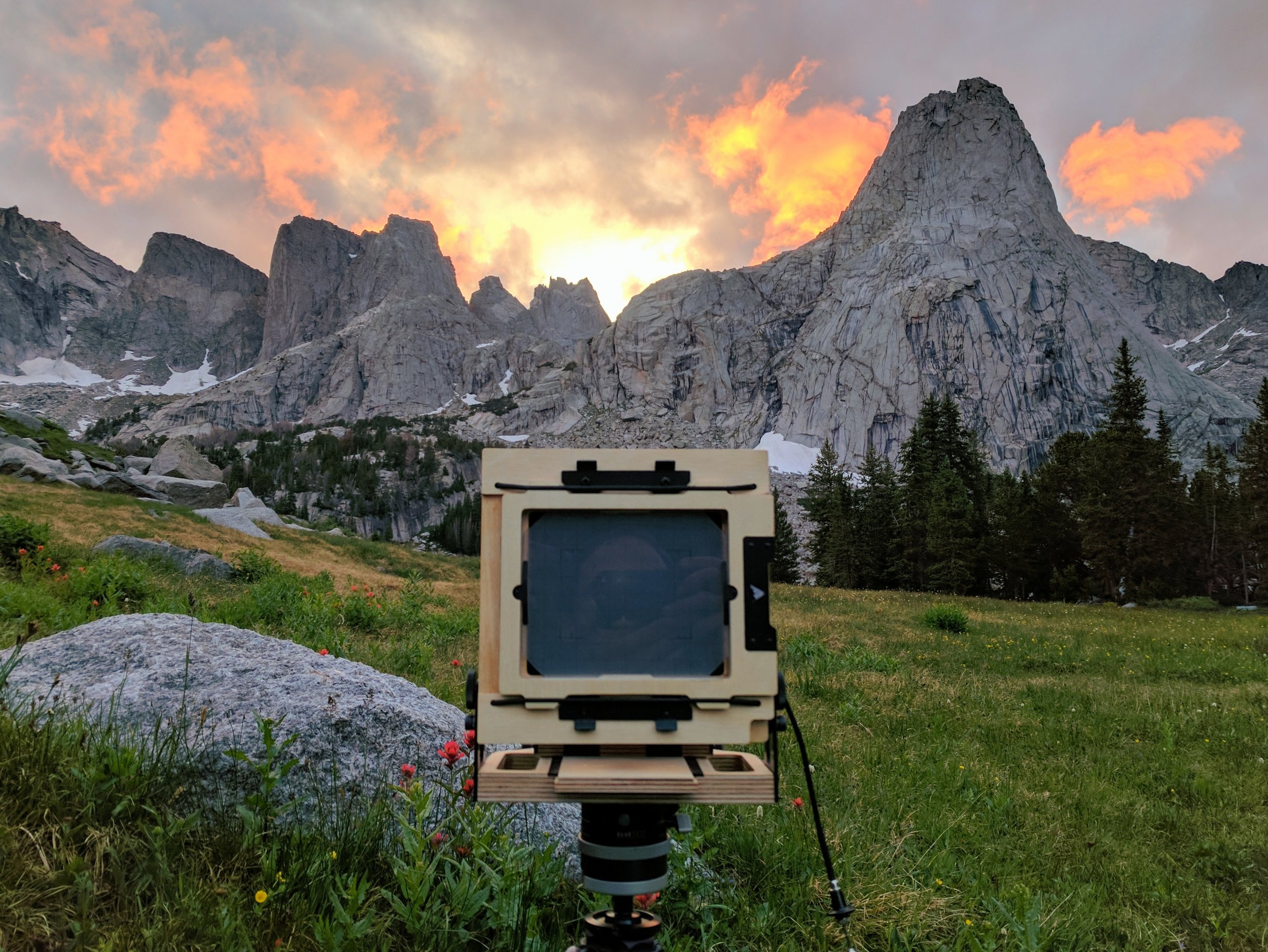This outdoor photograph captures a serene and colorful landscape at either sunrise or sunset. In the foreground, a lush, grassy area dominates the scene, showcasing vibrant green blades interspersed with patches of brown grass. Bright pink and yellow flowers add spots of vivid color among the greenery. Nearby, there's a sizable, flat, and grey stone partially embedded in the ground.

At the center of the image, a curious device stands out, featuring a beige, wooden-colored frame encasing a dark, charcoal black square that resembles a monitor or perhaps a camera lens. This device, with its electrical appearance and a port on the right side, hints at a potential use in photography or scientific measurement.

Beyond this grassy foreground lies a range of grey and cream-colored mountains, adorned at their base with evergreen trees that remain lush and green. The sky overhead is a stunning palette of colors, transitioning from light grey to rich orange and blue, likely illuminated by the rising or setting sun, casting a magical light over the tranquil scene.